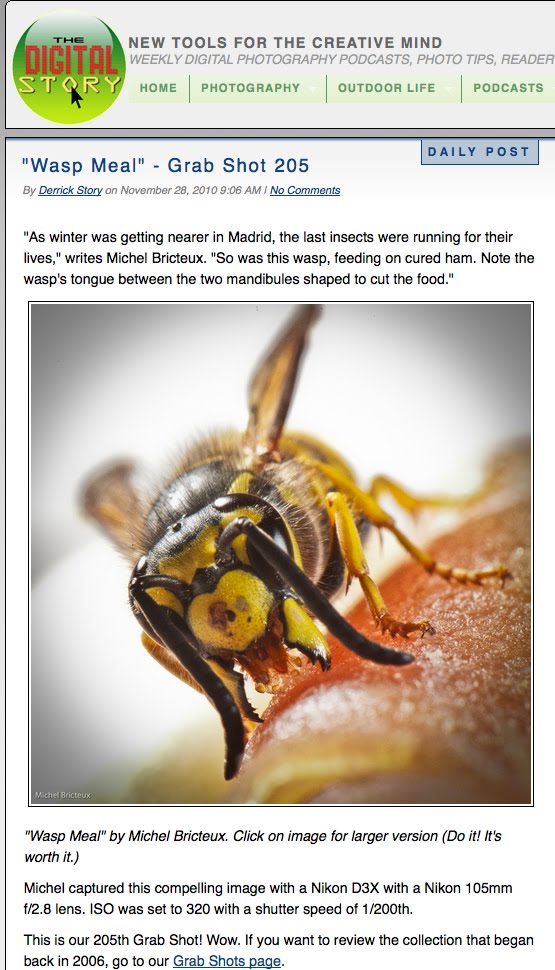A detailed caption that describes the image from the provided voice description might look like this:

---

This image is a screenshot of a website titled "The Digital Story," featuring a prominent banner that reads, "New Tools for the Creative Mind," and promotes a weekly digital photography podcast along with photo tips and more. At the top of the page, navigation links in green print are visible, including "Home," "Photography," "Outdoor Life," and "Podcast."

The main content area features an article titled "Wasp Meal," labeled as "Grab Shot 205" by Derek Story, dated November 28th, 2010, at 9:06 a.m., with no comments. On the upper right-hand corner, there's a section labeled "Daily Post," featuring a quote: "As winter was getting nearer in Madrid, the last insects were running for their lives," says Michael Bridestow. Below, it adds, "So was this wasp feeding on cured ham. Note the wasp's tongue between the two mandibles shaped to cut the food."

Accompanying the text is a large photograph of a wasp perched on a piece of ham, seemingly feeding. The caption below the image reads "Wasp Meal" by Michael Brideau. The text encourages viewers to click on the image for a larger version, asserting "Do it. It's worth it." Further details mention that Michael captured this compelling image using a Nikon D3X, followed by additional commentary about the photograph.

---

This caption encompasses all the pertinent details provided while organizing them into a coherent, informative description.